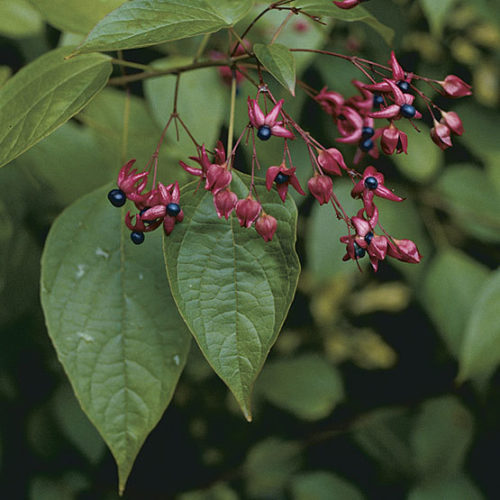This image showcases a close-up of a flowering plant with relatively thin branches. The plant's leaves, large given the slender stems, are shaped like water drops or elongated ovals with pointed ends. The focus of the image is on the striking flowers, which are deep purple with hot pink hues and possess blue, almost spherical centers resembling berries but not blueberries. The vibrant colors and intricate veins of the very green leaves are visible, with a smaller leaf in sharp focus showing water droplets, while larger leaves and more foliage blur into the background, creating a contrasting backdrop of various leaf shapes and sizes from different plants.